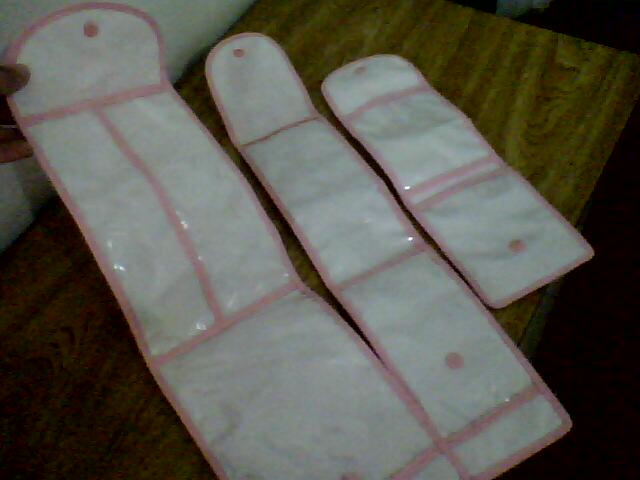The image captures three somewhat blurry plastic organizers, each with a white base and pink-lined edges. These organizers, which have a slightly reflective surface, are arranged on a dark brown wooden table or bench. The largest of the three is on the left and is being held by a hand visible in the top left corner, suggesting it might be actively examined. The middle organizer is moderately sized, while the smallest is on the right. Each organizer appears to feature pink buttons for closure and transparent sections, hinting at storage functionality, perhaps for items like shoes or travel essentials. The background includes a white wall, and the faint wood grain and shadow indicate an indoor setting. The flash from the camera is slightly visible on the plastic surfaces, adding to the overall clarity.